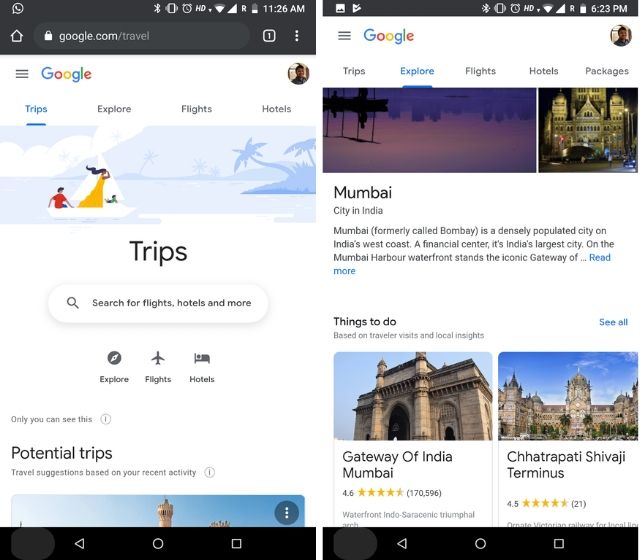**Detailed Caption:**

The image comprises two side-by-side screenshots from a Google phone, possibly a Pixel device. Both screenshots showcase the interface of Google Travel, with a distinctive black status bar at the top indicating the phone’s details such as battery level, Wi-Fi connection, and the time of day, all displayed in white icons.

**Left Screenshot:**

- **Header:** At the top, there is a search window displaying "google.com/travel".
- **Main Page:** Below the search window, the page has a clean, white background with the colorful Google logo prominently displayed.
- **User Icon:** Positioned in the upper right corner of the screen.
- **Graphic:** Central to the screen is an illustrated graphic depicting an island surrounded by the ocean with cartoon-like figures possibly representing people engaging in activities on the beach and in the water.
- **Title:** Center-aligned text saying "Trips".
- **Search Bar:** Directly under "Trips", there is a search bar with the placeholder text "Search for flights, hotels, and more" accompanied by a magnifying glass icon.
- **Navigation Icons:** Below the search bar, three icons labeled "Explore," "Flights," and "Hotels" appear, styled in black on white.
- **Partial Image:** At the bottom, it reads "Potential trips," followed by a partially visible image showing a blue sky and some architectural features.

**Right Screenshot:**

- **Header:** Similar details at the top with the white icons indicating the phone’s status.
- **Main Page:** The white-background Google page is visible, with the user icon again located in the upper right corner.
- **Menu Tabs:** The top section features text headers for navigation, including "Trips," "Explore," "Flights," "Hotels," and "Packages". The "Explore" tab is selected.
- **Images of Mumbai:** Beneath the headers, there are two images of the city of Mumbai, accompanied by a description paragraph detailing Mumbai.
- **Things to Do:** At the bottom, the section titled "Things to do" includes listings for attractions such as the "Gateway of India, Mumbai" and another option, both showcasing ratings of over four-plus stars.